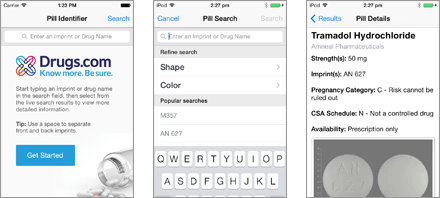The series of images show screenshots from an iPod capturing various stages of a drug identification search on Drugs.com. 

1. In the first screenshot, taken at 1:23 p.m., the user is seen on Drugs.com, attempting to identify a pill by entering its markings in the search field. The site prompt reads, "Enter imprint, drug name, or NDC." Due to the quality of the image, it's difficult to discern text beyond this point.

2. The second screenshot showcases the pill search interface. At the top, there’s an icon indicating pill search options where users can refine their search by shape or color. Popular searches listed include "M357" and "AN6...". Visible at the bottom is a standard QWERTY keyboard, suggesting that the user is about to enter further details or adjust the search criteria.

3. The final screenshot shows the results page. The pill in question is identified as Tramadol Hydrochloride with a strength of 50 milligrams and an imprint of "AN6...". Additional details include its classification under Pregnancy Category C, indicating that risk to the fetus cannot be ruled out, and its CSA Schedule N status, indicating that it is not a controlled drug. The pill is available by prescription only. 

The Drugs.com interface has a distinctive logo—a tall, hollowed-out 'X' with red, blue, pink, and dark blue squiggles—highlighting its unique branding. Through the series of screenshots, it is evident that the user successfully identified the pill as Tramadol Hydrochloride.